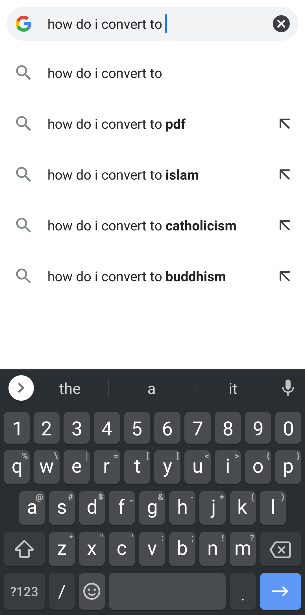The image depicts a screenshot of a cell phone displaying the Google website. At the top of the page, the familiar Google logo is visible, followed by a search bar with text partially entered, saying "how do I convert to". The input text is in black font, and the blue blinking cursor indicates the user is ready to continue typing. Below the search bar, Google’s autocomplete suggestions appear, each marked with a subtle diagonal arrow to the right. The first suggestion repeats "how do I convert to". The second option, in bold text, states "how do I convert to PDF". Following it, the next autocomplete suggestions read "how do I convert to Islam", "how do I convert to Catholicism", and "how do I convert to Buddhism", all in bold black ink. At the bottom part of the screen, a digital keyboard is prominently displayed, showing the interface through which the text was entered.